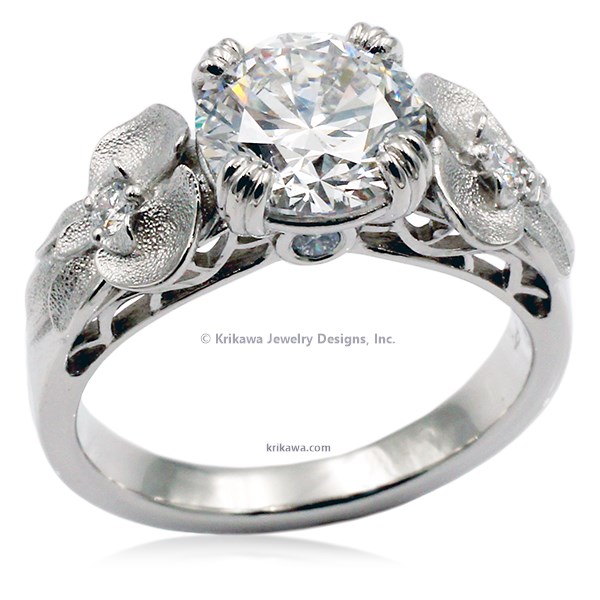This detailed product image, featuring an elegant engagement ring from Krikawa Jewelry Designs Incorporated, is captured on a completely white background, accentuating the ring’s exquisite details. The centerpiece of the ring is a large diamond, held in place by four prongs, which sparkles brilliantly under the bright lighting. Flanking the central diamond on either side are intricate, seemingly floral designs, each housing a smaller diamond at their core. The ring, which is either silver or white gold, displays a beautiful bumpy texture reminiscent of leaves or bows along its sides, further embellished with petite diamonds. The lower part of the band features delicate filigree work, allowing light to pass through and enhance the diamond’s brilliance. The high-angle three-quarter view of the photograph ensures all these fine details are visible. Central to the image is a small gray watermark reading "Krikawa Jewelry Designs Incorporated," and at the very bottom, just above the band, the website "krikawa.com" is displayed in fine print.